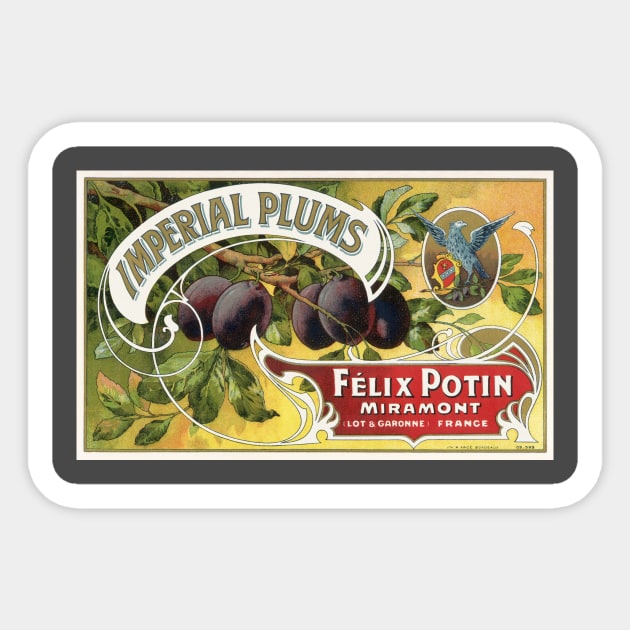The image is a detailed illustration, likely vintage, depicting "Imperial Plums." Central to the artwork is a branch adorned with lush green leaves and five dark purple plums, which are small, almost olive-like in size. The plums hang prominently from this single branch, which extends to the right side of the image. Surrounding this central imagery is a series of borders: a white border directly around the picture, enclosed by a black border, and then another white border.

Above the plums, in the upper right corner, there's a circle containing a blue bird with spread wings, perched on a branch. Adjacent to the bird is a gold badge featuring a red label and a blue bar, with some indecipherable black text beneath. At the bottom edge of the image, a red label in white text reads "Felix Potin, Miramont, Lot-et-Garonne, France," indicating a French company. The lid of what could be a container or sign is placed on a stark white surface, giving the impression of a historical yet elegantly designed product advertisement.